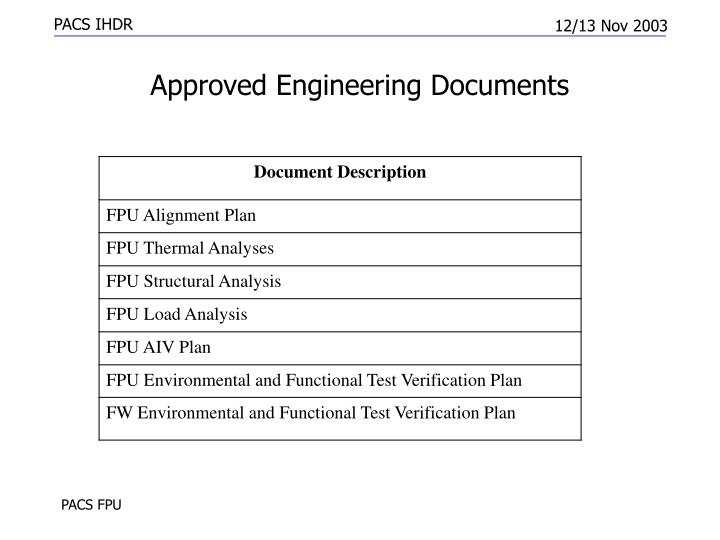The image depicts a formal document with a clean white background. At the top left corner, "P-A-C-S I-H-D-R" is written in black, uppercase letters. In the top right corner, the date "12/13 NOV 2003" is also displayed in black uppercase letters. Below these headings, a thin blue line separates them from the rest of the document. Underneath the blue line, the title "Approved Engineering Documents" is prominently positioned in black text. The central part of the document features a detailed table labeled "Document Descriptions." The entries within the table list several key documents: "FPU Alignment Plan," "FPU Thermal Analysis," "FPU Structural Analysis," "FPU Load Analysis," "FPU AIV Plan," "FPU Environmental and Functional Test Verification Plan," and "FW Environmental and Functional Test Verification Plan." Finally, in the lower left-hand corner, "P-A-C-S F-P-U" is inscribed in black, uppercase letters, consistent with the rest of the text.